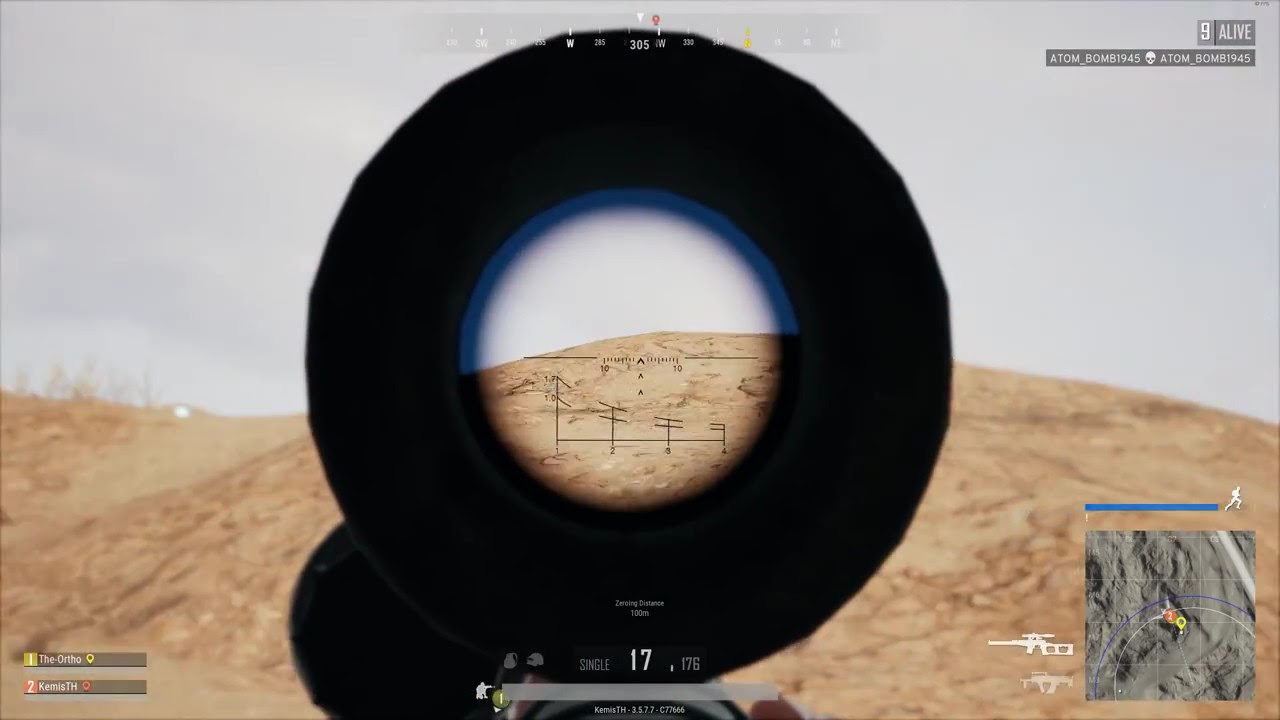This image is a color freeze-frame screenshot in a horizontal rectangular landscape orientation, depicting a scene that appears to be from a video game, looking through the lens of a sniper rifle scope. The background consists of a barren desert hill landscape with a gray sky overhead and some blurry patches of grass along a dirt mound at the bottom. 

In the center of the image is a large black circular object representing the scope, adorned with various digital readouts. Through the scope's lens, there's a visible numerical readout in the lower center showing the number "17" next to what appears to be an energy or power bar. Below this are numbered and dashed rulers, including the label "305 West." Additional text at the top reads "I live" and "atom bomb 1945."

In the lower right-hand corner, there is an inset close-up of the textured surface in gray, featuring a machine gun icon to the left. The lower left-hand corner displays player information: "The Ortho" assigned to player 1 and "Keenest TH" to player 2. Compass directions (SW, W, NW, N) are indicated near the top of the scope. Further numerical information about the rifle’s zoom or zeroing distance, set at 100, is also present. The image captures the detailed graphic elements typical of a video game interface.